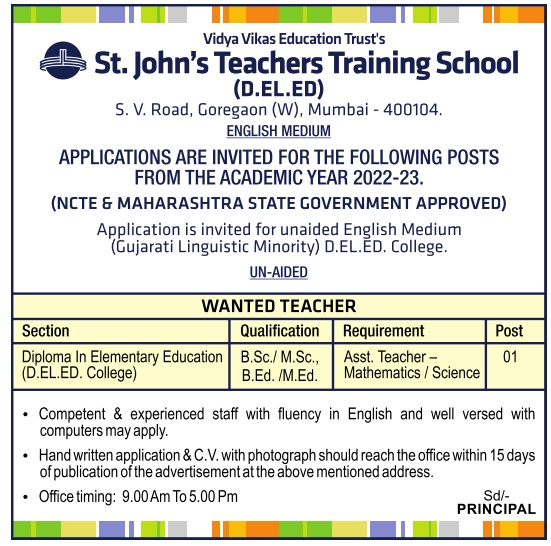The image captures an advertisement displayed on a bulletin board by the Vidya Vikas Education Trust, promoting St. John's Teachers Training School. The text on the ad reads:

"Vidya Vikas Education Trust
St. John's Teachers Training School (D.El.Ed)
S.B. Road, Gordagan, W. Mumbai 
English Medium

Applications are invited for the following post from the academic year 2022 to 2023. Approved by N.C.T.E. and Mariusta State Government, applications are invited for unaided English Medium positions. 

Wanted: Teacher
Section: Mathematics & Science
Qualifications: Diploma in Elementary Education (D.El.Ed)
Requirement: Bachelor's degree in Science (B.Sc)
Position: Assistant Teacher"

The ad specifies the need for a qualified assistant teacher in Mathematics and Science, with a proper mix of academic credentials and teaching certification.